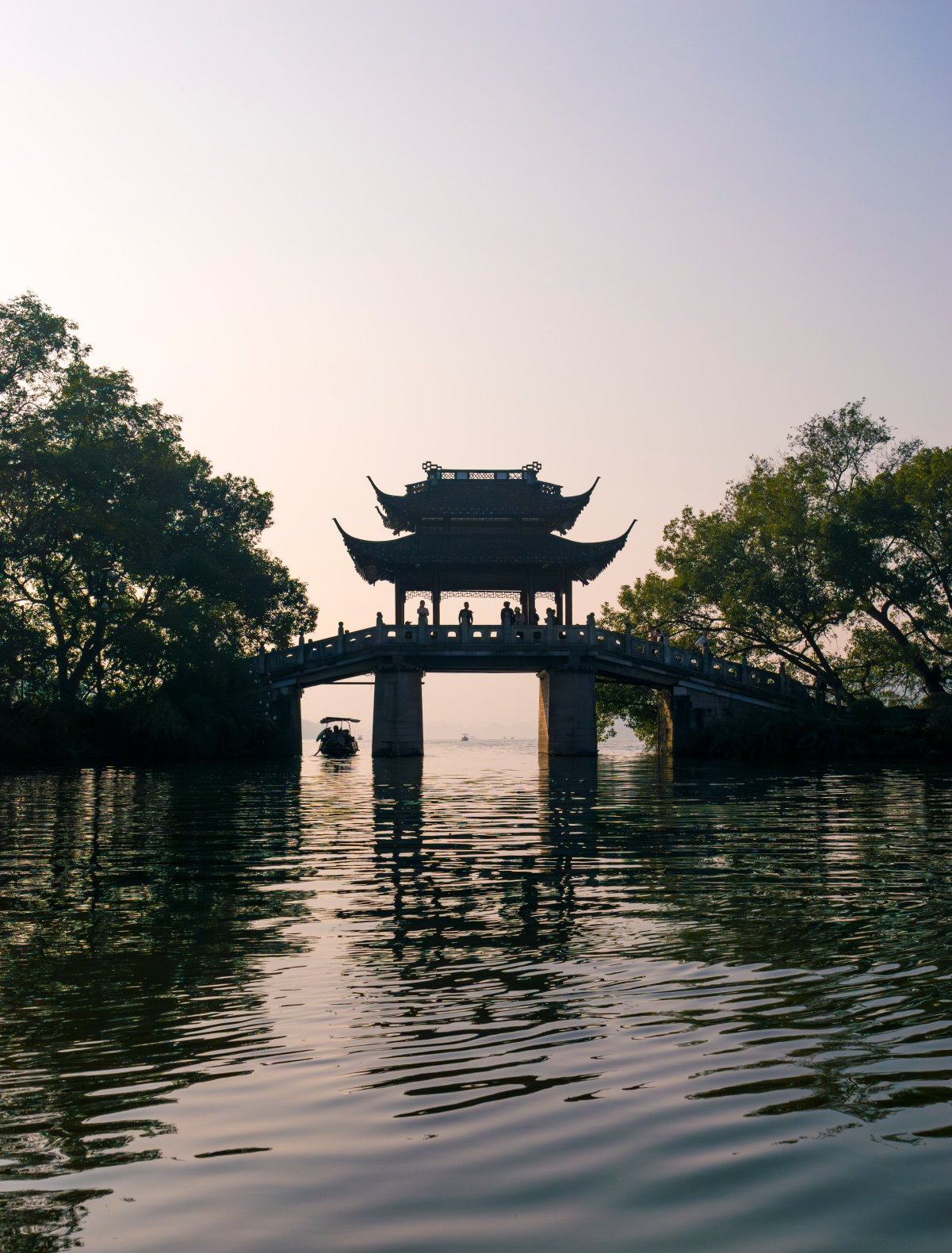The image depicts an Asian bridge over a body of water, possibly a lake or a river. The bridge features three distinct underpasses, with the middle one being larger and taller than the two narrower, shorter side ones. The structure arches upward, creating an elevated walkway that levels out in the middle and then descends. At the center of the bridge is an ornate canopy with traditional Asian architectural elements, such as upward-slanting edges that resemble the rooflines of houses or temples in Japan or China. The image is vertical, capturing the view from the water with the bridge framed by green trees on both sides. The sky transitions from a gray hue on the right to a pink-white on the left, suggesting a sunrise. The water below is a rippled blue-green, and in the shadow of the bridge, the silhouette of people can be seen standing and looking out. A boat with a small top can be seen through one of the underpasses, adding a tranquil, picturesque touch to the scene.